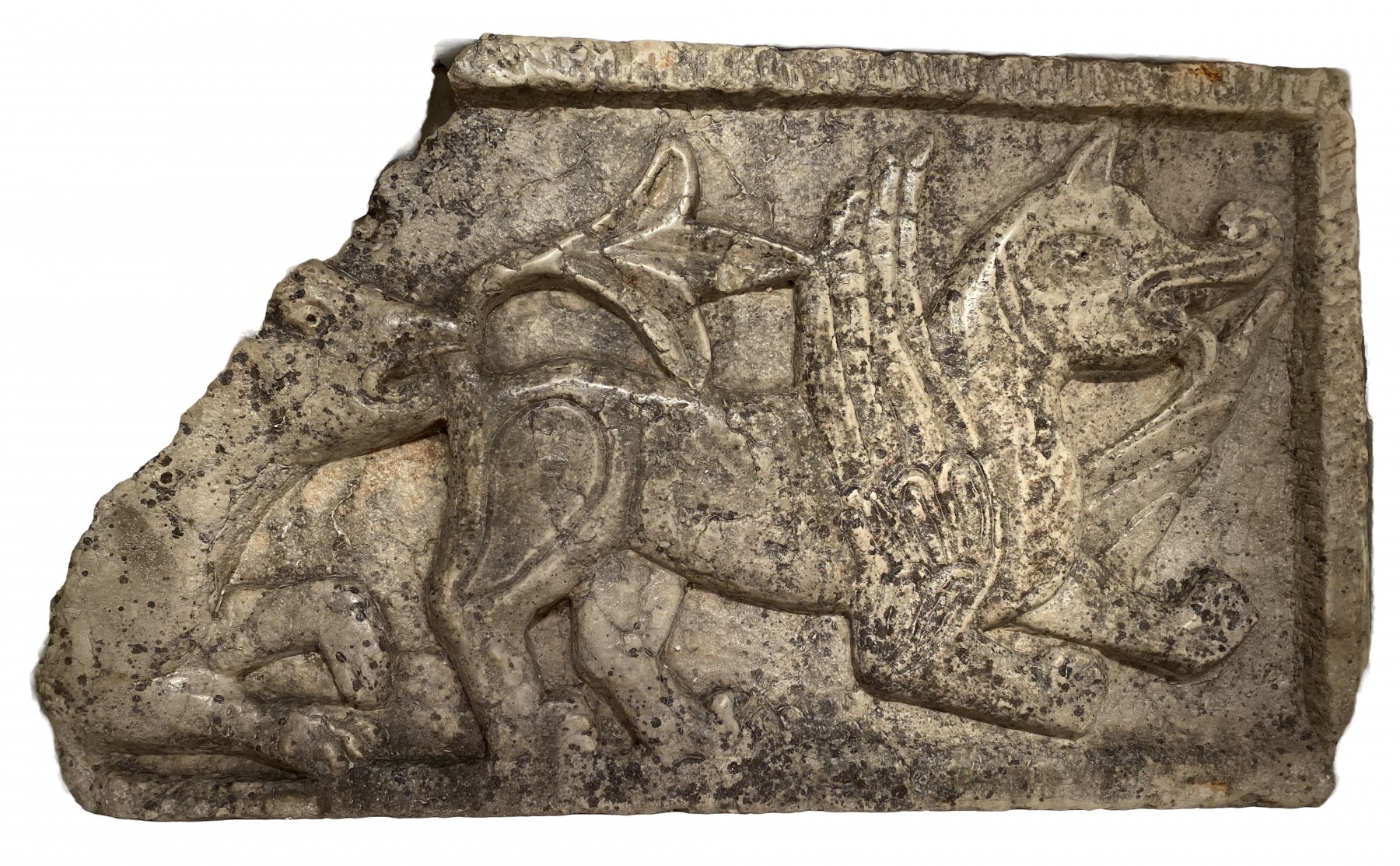This image showcases a detailed, aged stone slab, dominating its white backdrop, reminiscent of ancient artifacts seen in movies like Indiana Jones. The stone itself is dark gray, marbled with brown and light brown hues, interspersed with black speckles, suggesting significant age and weathering. The slab, appearing broken on the bottom right and left sides with jagged, diagonal cuts, hints at its antiquity.

Intricately etched into the center of the stone is an elaborate, winged creature with a fierce, open mouth and a tail that curls over its body. This creature, resembling a fantastical dragon or dog, appears to be fleeing to the right side of the slab. Accompanying it in the background is a smaller animal, shaped like a lizard with legs tucked under its body and its head angled upwards, seemingly nipping at the larger creature's hind end. The top and the remaining side borders of the slab are intact and well-formed, suggesting that the slab was once part of a larger structure, likely an ancient ruin or castle. This photograph could be capturing the slab for documentation, presentation, or exhibit purposes.